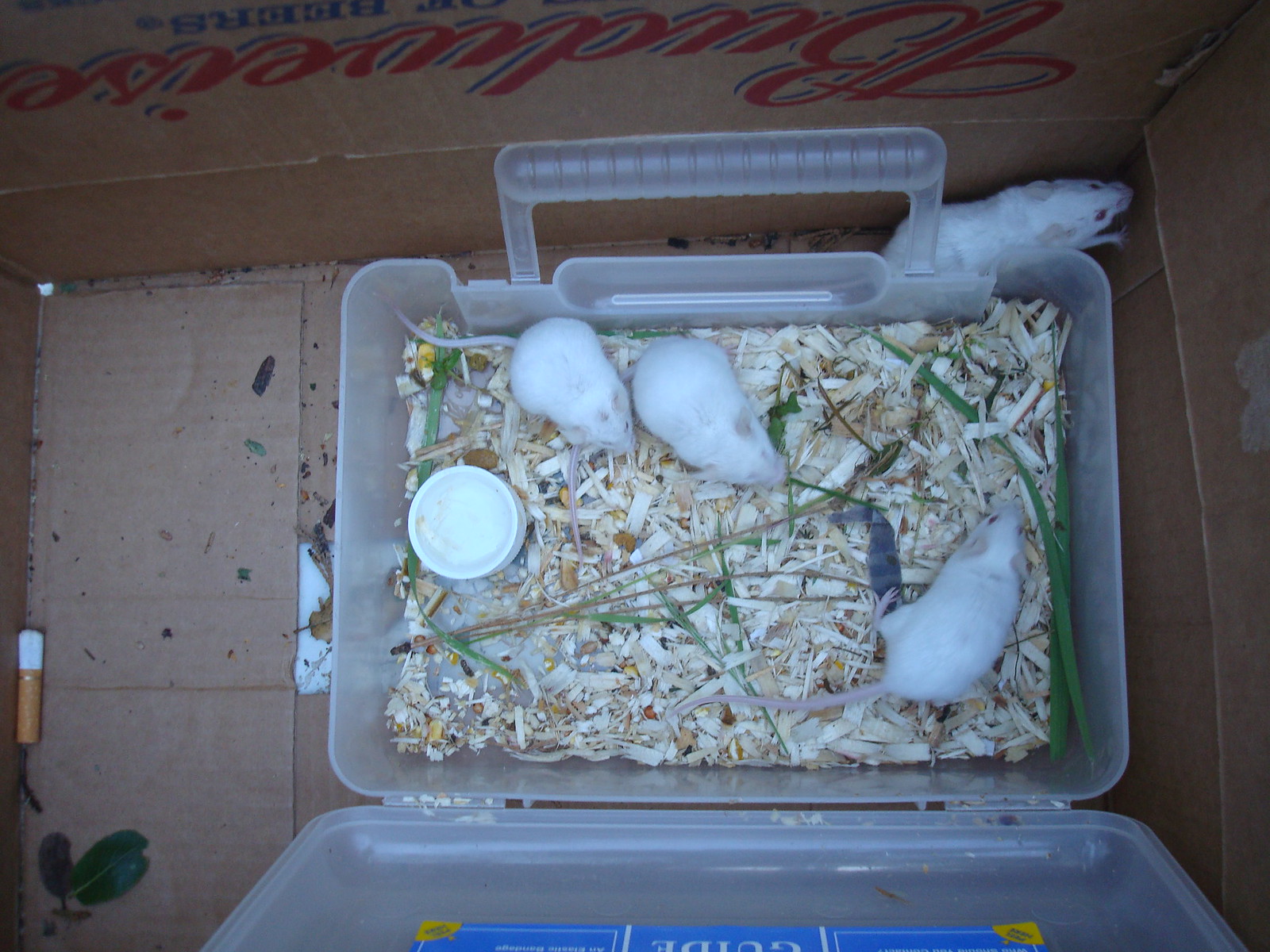The photograph is taken from a top-down perspective, looking into an open cardboard box bearing the red script logo of Budweiser upside down at the top edge. Inside this larger box, there is a clear plastic container with a handle, resembling a lunchbox, whose lid is open and extends out of the frame. The plastic container holds three white mice with red eyes sitting amongst a bed of light brown and beige wood shavings or straw, providing them with a makeshift surface. Inside this container, there is also a small pot, possibly for food or water, along with scattered seeds and some greenish plant material.

One additional white mouse is outside the plastic container, positioned in the top right corner between the plastic case and the cardboard box. The surrounding cardboard box contains some miscellaneous debris, notably a dark green leaf and a partially smoked cigarette butt on the left side. The scene captures a curious and somewhat cluttered environment for the mice.